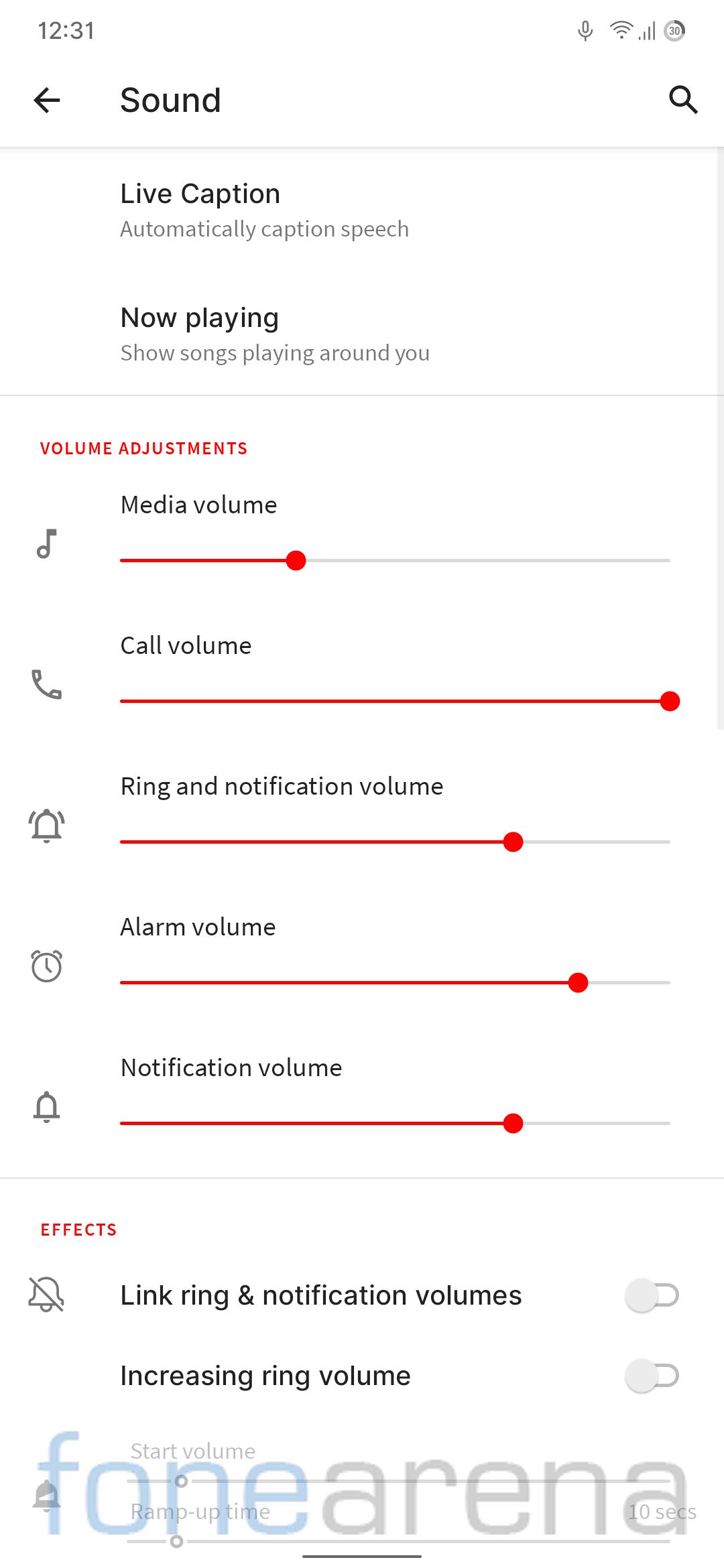The image displays a screenshot of a smartphone's sound settings interface, clearly watermarked by Phone Arena. At the top, the interface features categories such as "Live Caption," "Now Playing," and "Volume Adjustments." Detailed sliders in red allow for the adjustment of different audio levels including media volume, call volume, and ring notification volume. Notably, the option for increasing ring volume is turned off. All text throughout the interface is presented in black, with the exception of the word "Effects," which is highlighted in red. The status bar at the top of the screen indicates the time as 12:31, shows full Wi-Fi connectivity, and a fully charged battery. This image provides a comprehensive look at the detailed customization options available in the sound settings on this particular smartphone.